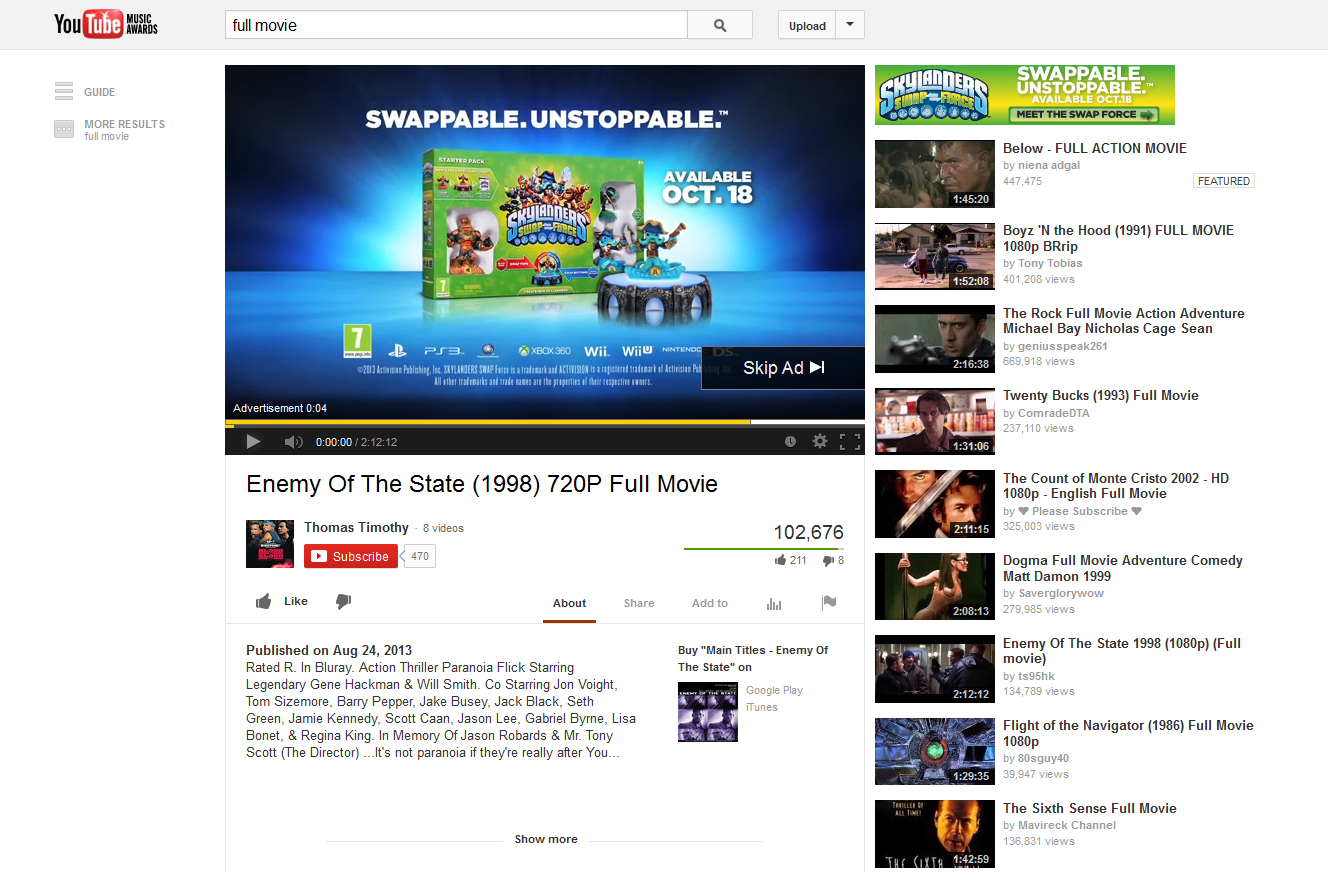The image showcases a YouTube webpage with the classic logo, where "You" is displayed in black letters next to "Tube" in white letters, all encased in a red box. The user has typed "full movie" into the search bar and is currently viewing an advertisement before the film starts. The ad, which promotes a new game available on Wii titled "Skylanders," declares itself as "swappable, unstoppable," and indicates availability starting October 18th. The user has the option to skip the advertisement, but it’s nearly finished as evidenced by the gold progress bar moving towards the right.

Below the ad, the main content area displays the full movie "Enemy of the State" from 1998, which was uploaded on August 24th, 2013. The description of the movie is visible along with related information. To the right of this section, the ad reiterates its message of being "swappable, unstoppable," and prominently features the "Skylanders" game. The sidebar provides a selection of full-action movies, each accompanied by still images from different scenes to help viewers decide if they might enjoy them.